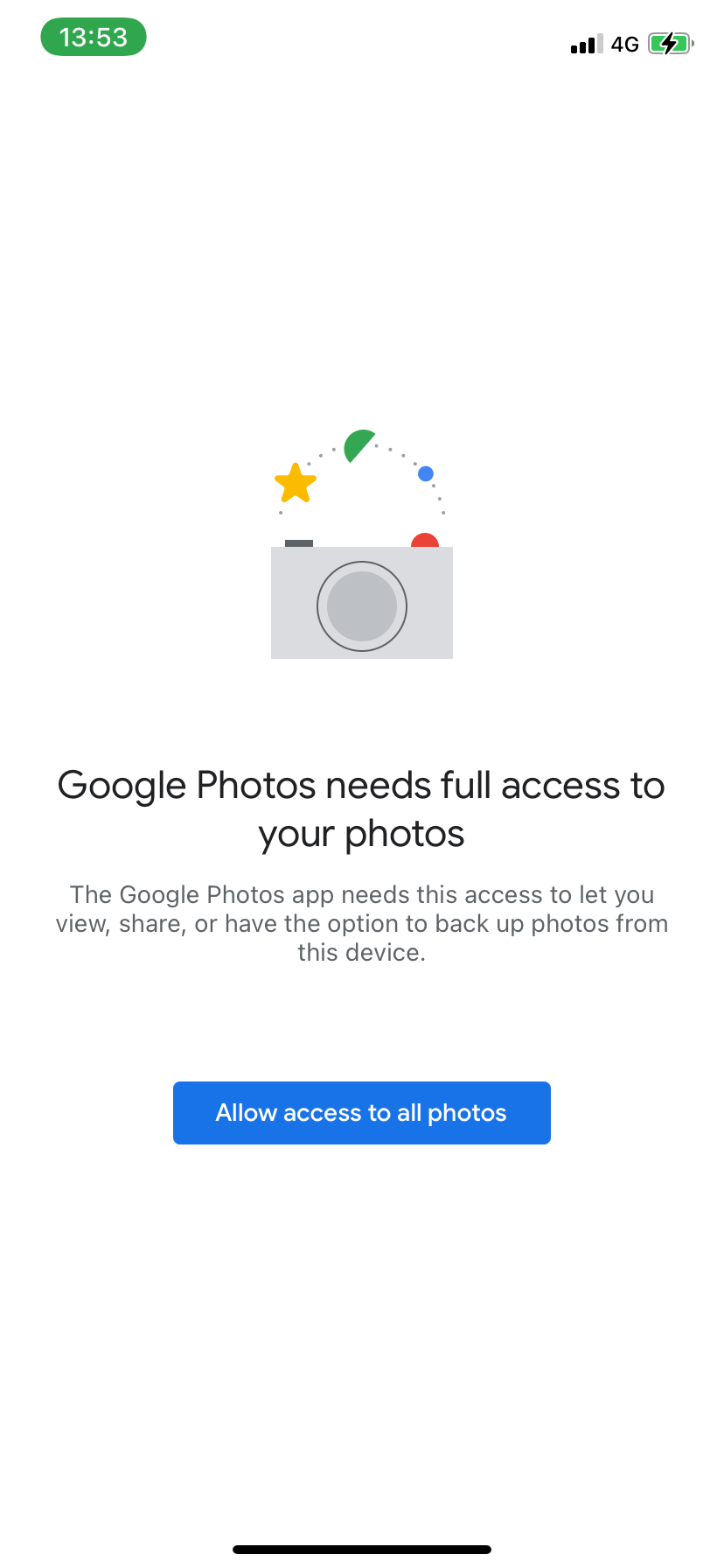The image shows an access permission page for Google Photos displayed on a smartphone. At the top left corner of the screen, the time is shown as 13:53 within a green capsule shape with white text. On the top right, there are four signal bars, the "4G" label indicating the network, and a nearly full battery icon displayed in green with a lightning bolt symbol over it, signifying that the phone is charging.

In the center of the screen, an illustrated camera icon is depicted in gray, adorned with a yellow star, a green half-circle, a small blue circle, and a red circle, all interconnected by an arched, dotted circular shape. Below this icon, a message in thin font reads: "Google Photos needs full access to your photos," followed by a more detailed explanation in gray text: "The Google Photos app needs access to let you share, view, and have the option to back up photos from this device."

Further down, there is a significant amount of white space leading to a large rectangular button with curved corners. This button is medium bright blue and features white text that reads: "Allow access to all photos." The bottom of the phone has a small, thin black line, about four or five pixels in height, centered across the base. The layout prominently features a considerable amount of white space both above and below the text, with all content centrally justified.